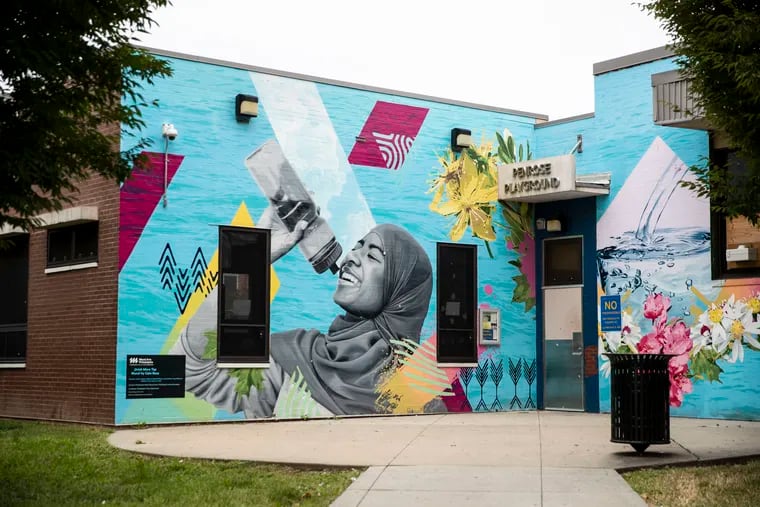The image depicts the front of a brick building, identified by a sign above the entrance as "Penrose Playground." The photo is taken at an angle, showcasing a concave corner where two walls meet. Both walls feature a predominantly light blue mural with various decorative elements, including flowers, purple rhombus-shaped designs, and a large depiction of a young woman in a tunic or hijab drinking from a sport bottle. The scene exudes a water theme, with water imagery evident across the mural, including water being poured into a container. Dominating the top of the image is an overcast, white sky. In the upper left, branches of a tree are visible, adding a natural touch. The building is bordered by a gray concrete sidewalk leading to a circular walkway in front of the metal door, which has an awning-like sign above it. The green grass flanks the sidewalk, and a trash can mounted on a single post stands to the right near the door. The overall atmosphere captures an outdoor, community-friendly space with artistic and natural elements combined.